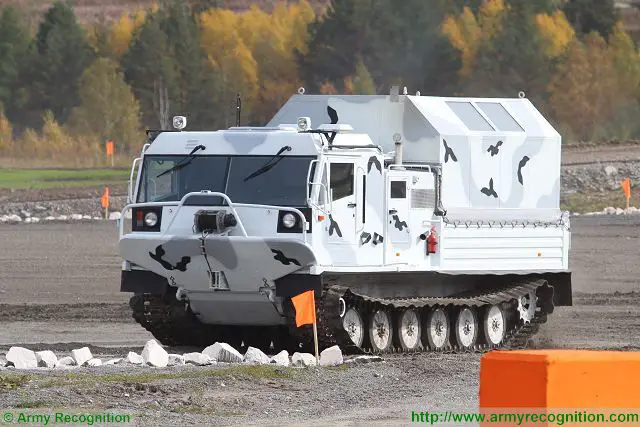This is a detailed photograph of a white military tank with black and gray camouflage patterns, captured on a flat, gray ground. The tank features a total of seven gears on each side, connected by a gear chain to its track tires, which enable it to traverse various terrains. The tank has a dominant, boxy, armored look with a large tinted windshield taking up almost the entire front surface, accompanied by two downward-hanging windshield wipers. A coiled pulley system is hooked underneath the grille at the vehicle’s front. On top of the cabin is a spotlight, and there are additional design elements like a black, three-winged stamp on different parts of the tank. 

The bottom left corner of the photo bears the green-printed copyright symbol and "Army Recognition," while the lower right corner displays the URL "http://www.armyrecognition.com" in similar green print. In the background, a forest with trees displaying various shades of green and autumn colors can be seen, though slightly out of focus. The tank is traveling on a dirt path, marked by rows of white stones and multiple orange flags, suggesting it is in a designated practice area. There are also indications of multicolored trees further back. The tank takes up a significant portion of the image, positioned centrally and occupying nearly half of the photo, which is rectangular and in landscape view.